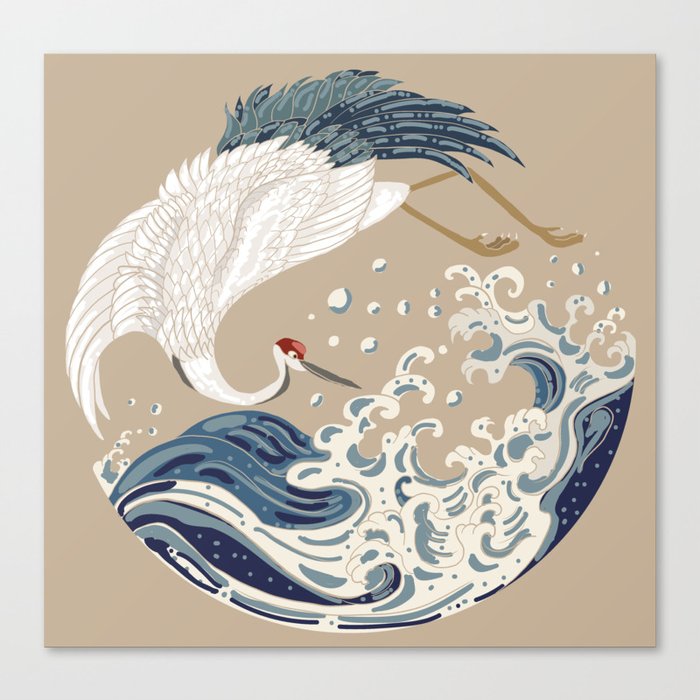The image is a detailed illustration, slightly taller than it is wide, with an off-white background framing a central beige square, inside of which an intricate painting unfolds. The painting, reminiscent of a Japanese woodblock style, features a circular composition formed by a crane and a wave. The crane, depicted with white feathers and a red-capped head, has a long, pointy gray beak and light brown talons extending to the right. The bird's gracefully curved neck and body create a semicircle, its dark blue and gray tail feathers arching up and to the right. The scene also showcases a dynamic wave in the bottom right, represented with shades of blue ranging from light to dark, and highlighted crests in light blue. This swirling water complements the crane, completing the circle-like design, evocative of the yin-yang symbol. The artwork is accentuated by subtle shadows along the right and bottom sides, adding depth to the composition.